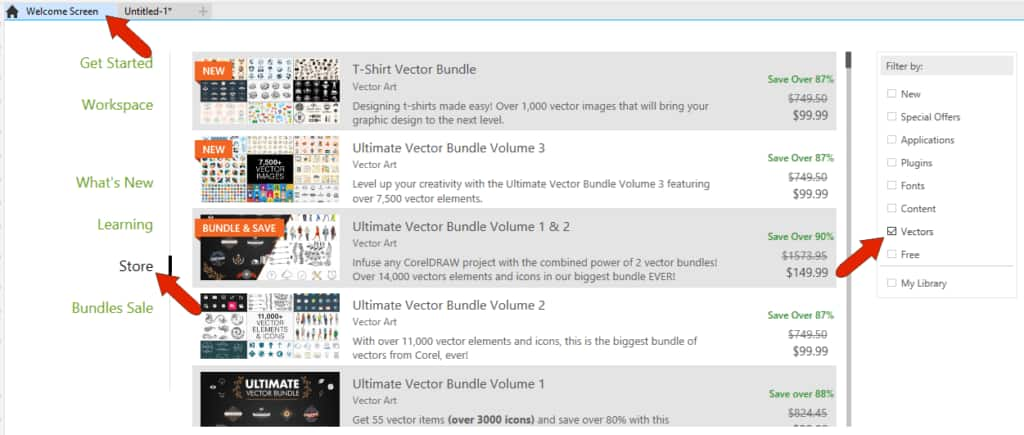The website's interface is detailed in this image. At the top of the webpage, a gray banner frames the content. Above it lies a small blue section with the text “Home” and “Welcome Screen” in black font. A red diagonal arrow originates from the white lower part of the image, pointing upwards towards the text, indicating attention. Adjacent to this, within the gray banner, is the title “Untitled 1” followed by a blue line.

On the left sidebar, a vertical menu displays categories such as "Get Started," "Workspace," "What's New," "Learning," "Store," and "Bundle Sale." These options are listed in light green text, except for "Store," which is in black text with an upward-pointing arrow. Below it, a segment alternates between gray and white backgrounds, presenting bundle items. 

1. The first item named “T-shirt Vector Bundle” focuses on vector art.
2. It is followed by “Ultimate Vector Bundle Volume 3.”
3. Next is “Ultimate Vector Bundle Volume 1 and 2.”
4. The fourth item is “Ultimate Vector Bundle Volume 2.”
5. Finally, “Ultimate Vector Bundle Volume 1” is listed.

Each item details savings, the price, and the sale price.

On the right side of the page, a rectangular filter panel presents sorting options, with squares for selection beside each category. These categories include "New," "Special Offers," "Applications," "Plugins," "Fonts," "Content," "Vectors," "Free," and "My Library." The "Vectors" category is selected, highlighted by a thick red arrow pointing at it.